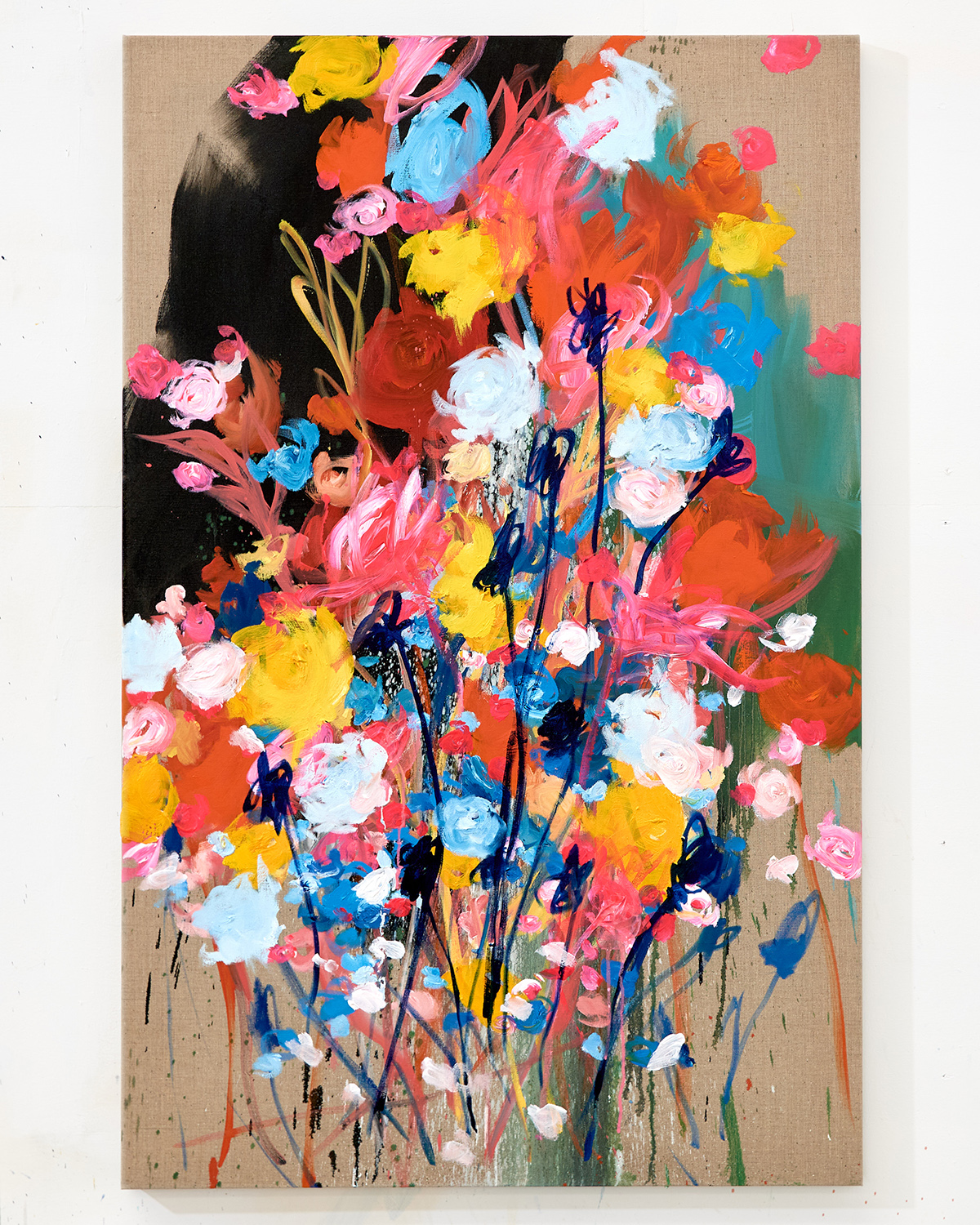The image features a light brown background accentuated by a prominent dark brown streak. At the forefront, a vibrant and abundant assortment of flowers showcases a dazzling array of colors, including pink, white, orange, yellow, blue, and striking red blooms. The flowers appear chaotically arranged, with their blossoms turned in various directions, creating a sense of natural wildness and spontaneity. Scattered among the floral display are delicate blue stems and a few green leaves, adding depth and contrast. Additionally, the composition is punctuated by bold blotches of blue and green, further enriching the visual tapestry. The scene is a rich explosion of color and texture, capturing a vivid and dynamic celebration of floral beauty.